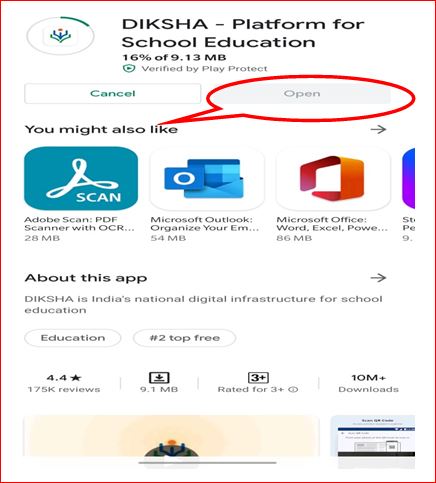The image is a screenshot framed by a thin red border, forming a large square. Inside this square, the background is black with gold accents. Prominently displayed in all capital letters is the word "DISK," followed by "SEJ, Platform for School Education." Below this text, it indicates a download progress of "16% of 9.13 megabytes."

There is a prominent circular message bar pointing towards a section labeled "You might also like," which includes options to "Cancel" or "Open." Beneath this, there are further options for "Scan," "Microsoft Outlook," and "Microsoft Office." Below these options, there's a section titled "About this app" with an arrow pointing to the right.

Additionally, there's an informative note stating, "DISKA is India's National Digital Infrastructure for School Education." Further down, there are buttons or bubbles displaying category rankings and ratings: "Education," "Number 2," "Top 3," accompanied by a user rating of "4.4 stars" from 875,000 reviews.